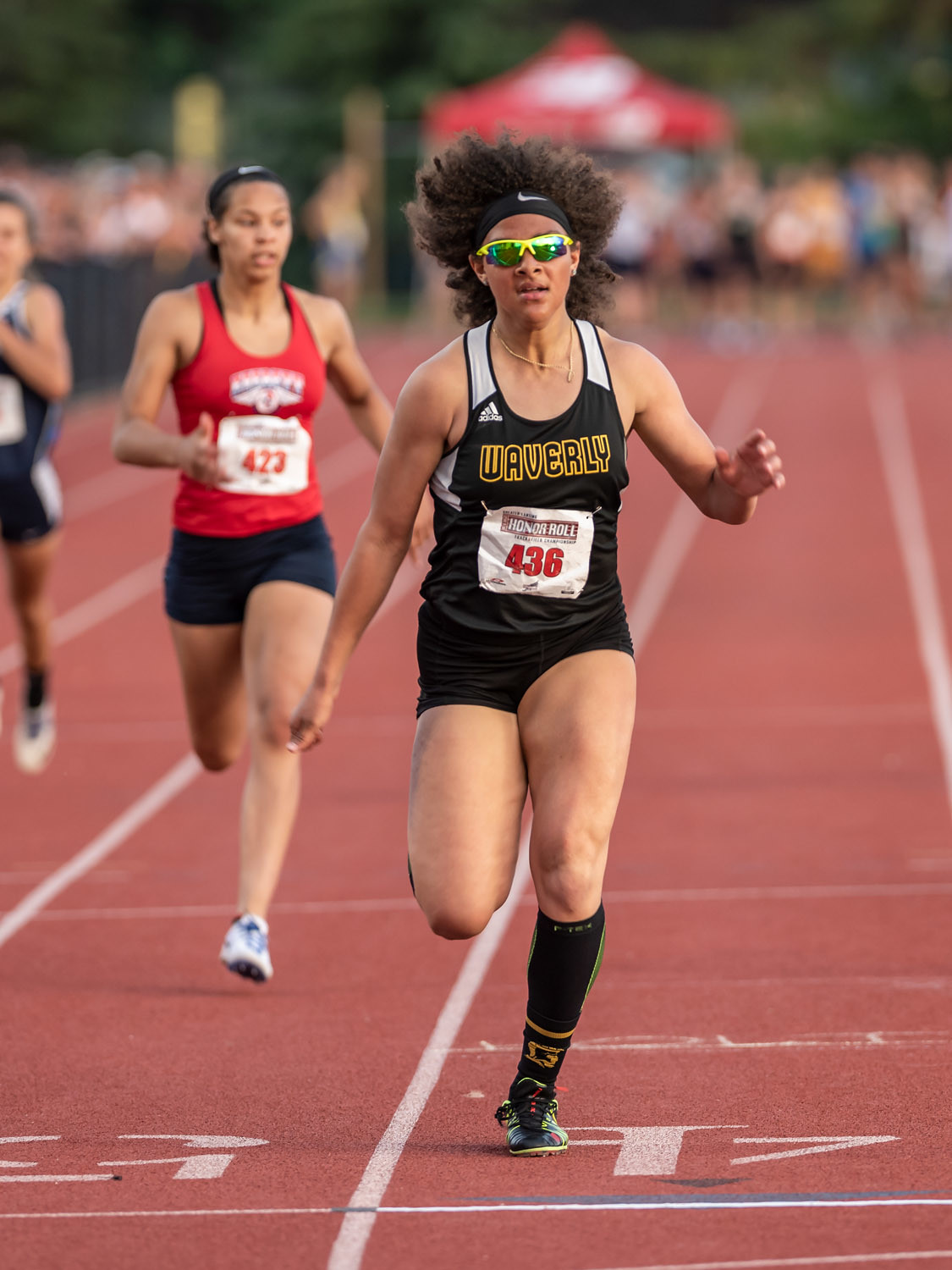The image captures a dynamic and intense moment of a track event with a focused and determined female athlete at the center. The main runner, a Black woman with tight, curly hair pulled back by her rapid pace, is wearing distinctive yellow-trimmed sunglasses and a black headband. Her athletic attire includes a black tank top emblazoned with "Waverly" in yellow letters, paired with black shorts, and complemented by long black socks and running shoes. The track beneath her feet is a vibrant red with white markings, indicative of a professional competition setting. Pinned to her chest is racer number 436, clearly visible as she sprints forward. Two other competitors trail behind her, slightly out of focus. One, wearing a blue tank top and black shorts, and the other, closer to the foreground, dons a red tank top with white shoes. The blurred background suggests it's a bright day, adding to the vividness of this exhilarating athletic moment.